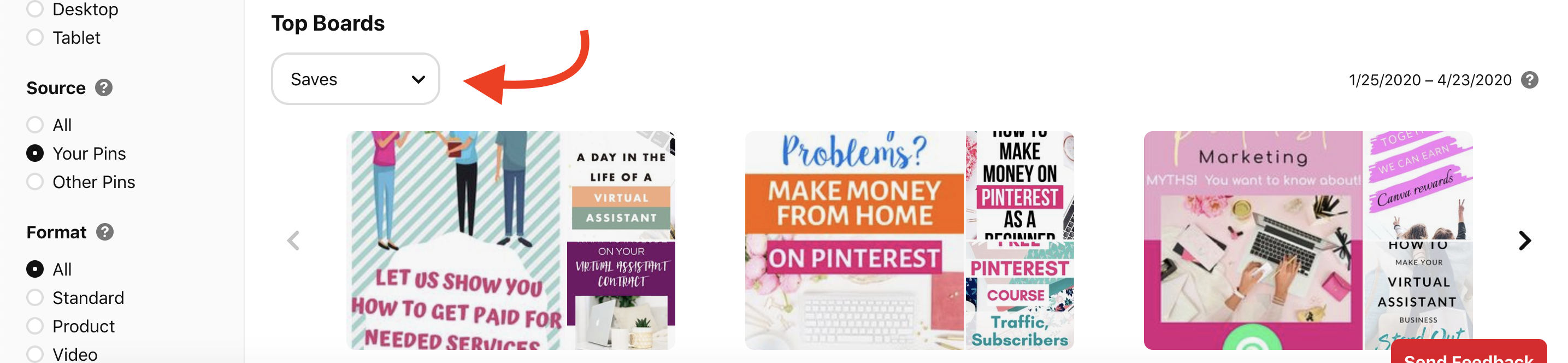This image is a partial screenshot captured from a Pinterest page interface. The left side of the screenshot features a vertical light gray sidebar with various filter and view options, including selections for desktop, tablet, and source, as well as format preferences. The 'source' option is currently set to 'your pins' and the 'format' set to 'all.' 

On the right side, against a clean white background, there is a prominently displayed heading in black that reads "Top Boards." At the bottom of the page, three square thumbnail boxes are aligned horizontally, each showcasing different types of Pinterest pins. The first thumbnail on the left highlights a pin about "how to get paid for needed services." The middle thumbnail features a guide on "how to make money from home on Pinterest." The rightmost thumbnail is labeled "marketing," completing the neatly organized visual presentation of the pins.